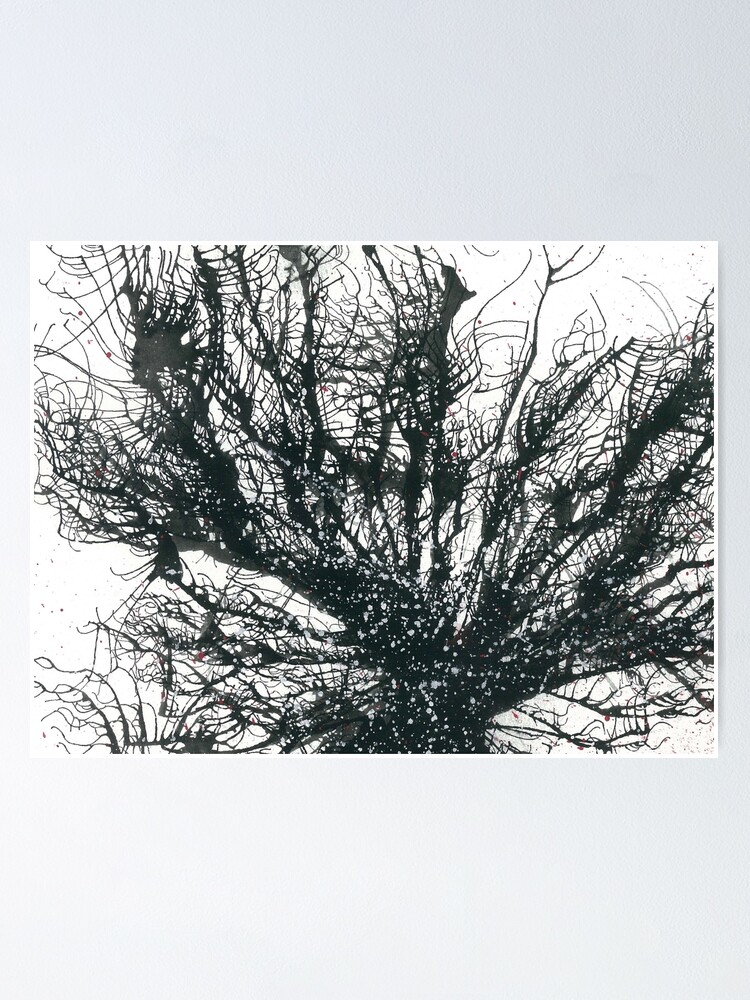The image depicts a contemporary piece of art resembling a tree with intricate black ink lines forming the trunk and sprawling branches. The branches extend outwards from the center, creating a complex, almost chaotic pattern. Highlights of red dots are scattered intermittently across the image, reminiscent of paint sprinkles from a brush. The background transitions from a grey gradient at the top to almost white at the bottom, complementing the white border surrounding the central figure. This could be interpreted as snow on the branches, enhancing the intricate design further. The artwork's white background allows the detailed network of lines and occasional red splotches to stand out, giving the entire piece a surreal and dynamic look.